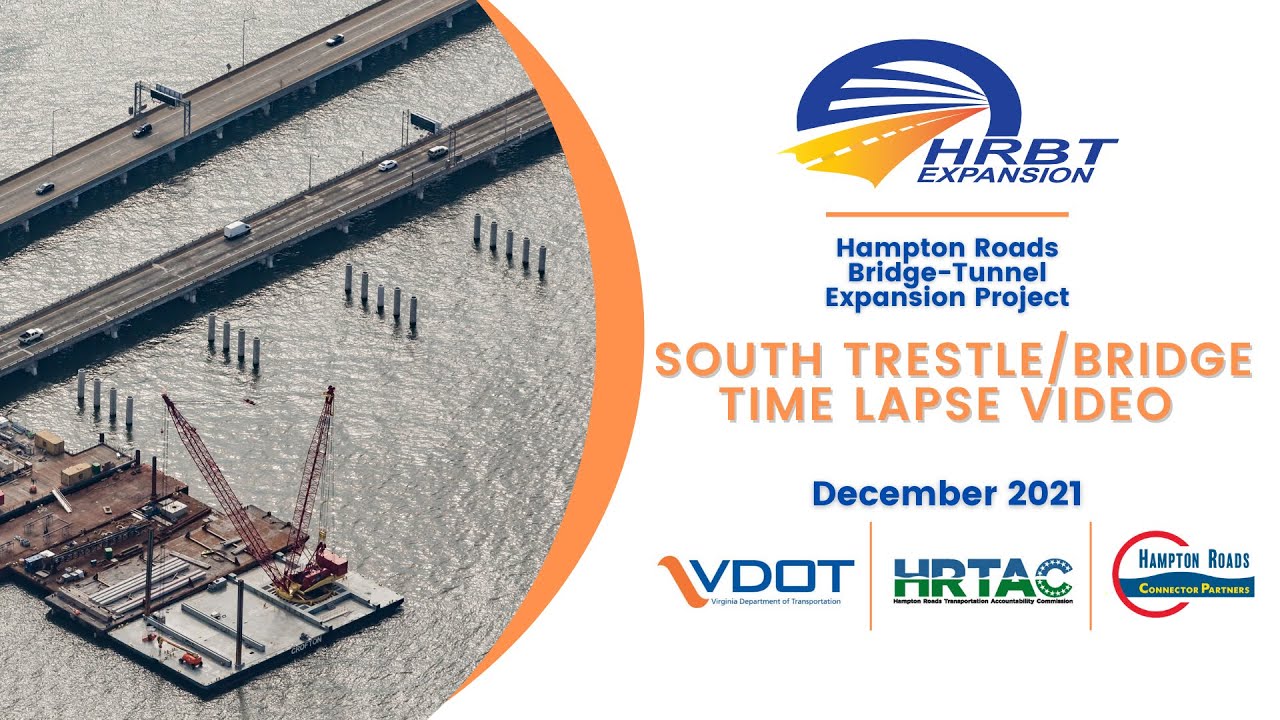The advertisement showcases the Hampton Roads Bridge Tunnel (HRBT) Expansion Project. The HRBT Expansion logo, prominently displayed in the upper right corner, features a blue tunnel with an orange road disappearing into it. Beneath the logo, the full name "Hampton Roads Bridge Tunnel Expansion Project" is written, followed by the title "South Trestle Bridge Time Lapse Video, December 2021." 

To the left, within a circular frame resembling a camera lens view, there is an overhead shot of the South Trestle Bridge and its surroundings. This image captures the trestle bridge being disassembled by numerous barges equipped with cranes, indicative of preparatory work for the HRBT Expansion. The scene includes two parallel bridges, each carrying two lanes of traffic—one for each direction. Cars are visible on both bridges, traversing over what appears to be a large body of water, possibly part of a harbor, with poles sticking out of the water. 

The sponsors for this project—VDOT (Virginia Department of Transportation), HRTAC, and Hampton Roads Connector Partners—are listed at the bottom of the ad. The imagery and text seem to imply that viewers can click to watch the time-lapse video of the South Trestle Bridge’s progress.